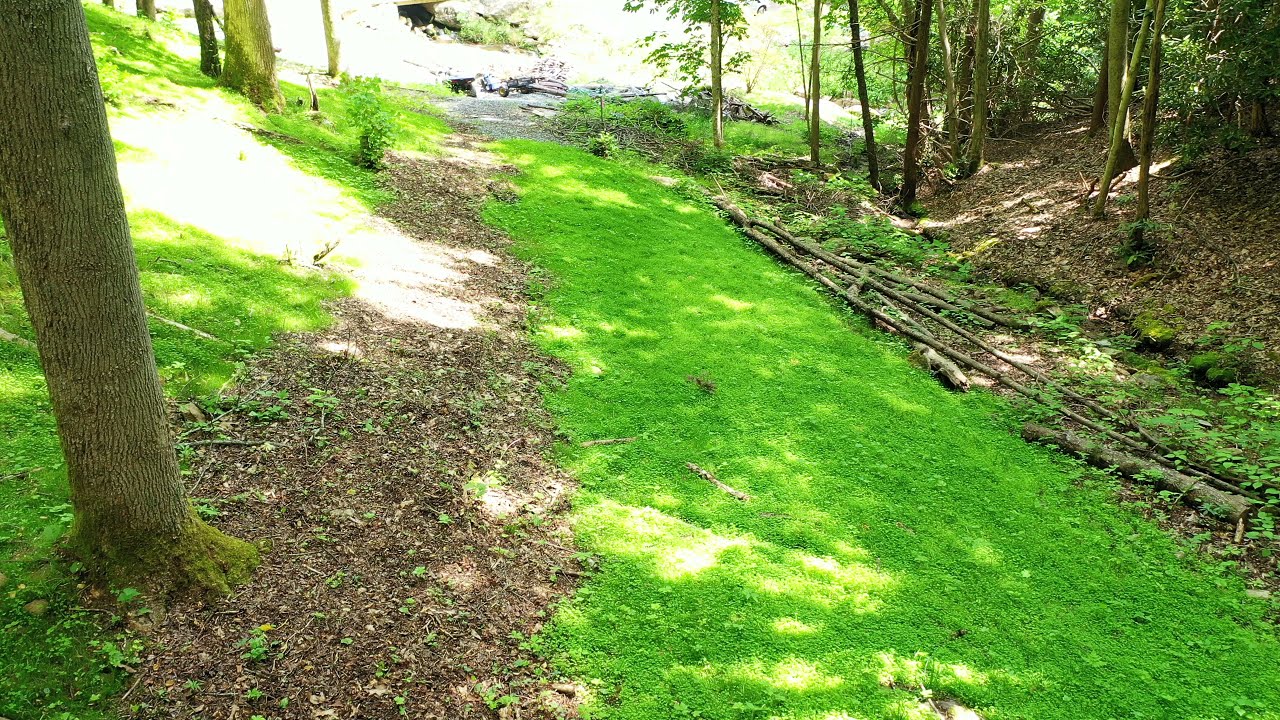The image captures a tranquil pathway in a vibrant park setting, enveloped by lush greenery on either side. The path itself is mostly dirt with sporadic patches of sparse green plants. To the left of the path, green grass thrives alongside patches of dirt, and near the bottom left, a tree trunk reaches upward, adorned with moss at its base. In the foreground to the right, several narrow, thin logs lie scattered on the ground. The top right of the image shows slender tree trunks with green plants visible in the background. Light filters through the trees, casting bright patches on the ground, contributing to a serene yet dynamic natural setting, devoid of any people or man-made structures. The background hints at a possible incline on both sides, suggesting a valley-like appearance. There are also indications of a gravel-paved area with some vehicles faintly visible in the distance.